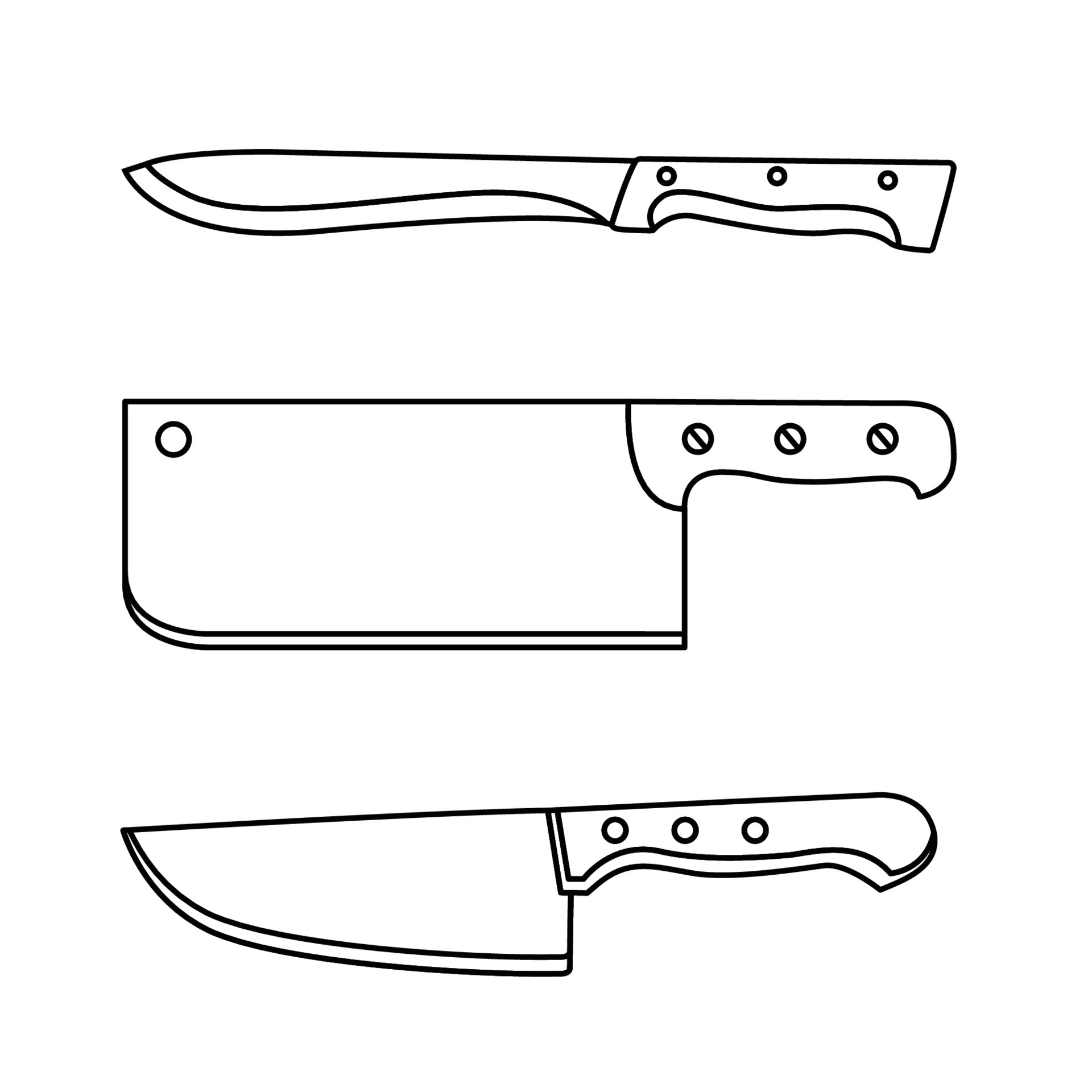This image features a black-and-white rendering of three distinct kitchen knives, all drawn with simple hand-drawn outlines devoid of color. 

At the top, there is a standard butcher knife with a slightly curved, thin blade and a riveted handle that includes a grip guard for added safety. The middle knife is a cleaver with a notably wide and thick blade, including a hole at the top left corner of the blade for hanging. Its handle is larger, secured with screws, and features a finger guard at the bottom. 

The bottom knife is a French knife, also known as a bread knife, it has a wide blade with a pointed tip. Like the first knife, the handle is riveted. All three knives are oriented with the blades pointing to the left and the handles to the right, against a plain white background, emphasizing their simple yet detailed line drawing presentation.